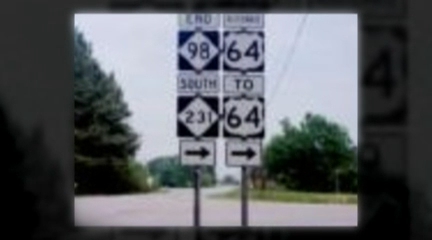This image showcases two vertical columns of road signs mounted on silver poles. The left column features a series of white diamond-shaped signs with black text. From top to bottom, the signs display "End 98" and "South 231," accompanied by an arrow pointing to the right. The right column, though less clear at the top, includes a shield-shaped sign indicating "64" at the top, followed by a square box with the number "2," another shield-shaped "64" sign, and an arrow pointing to the right.

The photograph is taken during the daytime, capturing a road in the background alongside multiple large shrubs. The style of the image suggests it may be a photograph superimposed on another, contributing to its overall blurriness. Minimal additional details are discernible, except for a faint power line running underneath the signs.